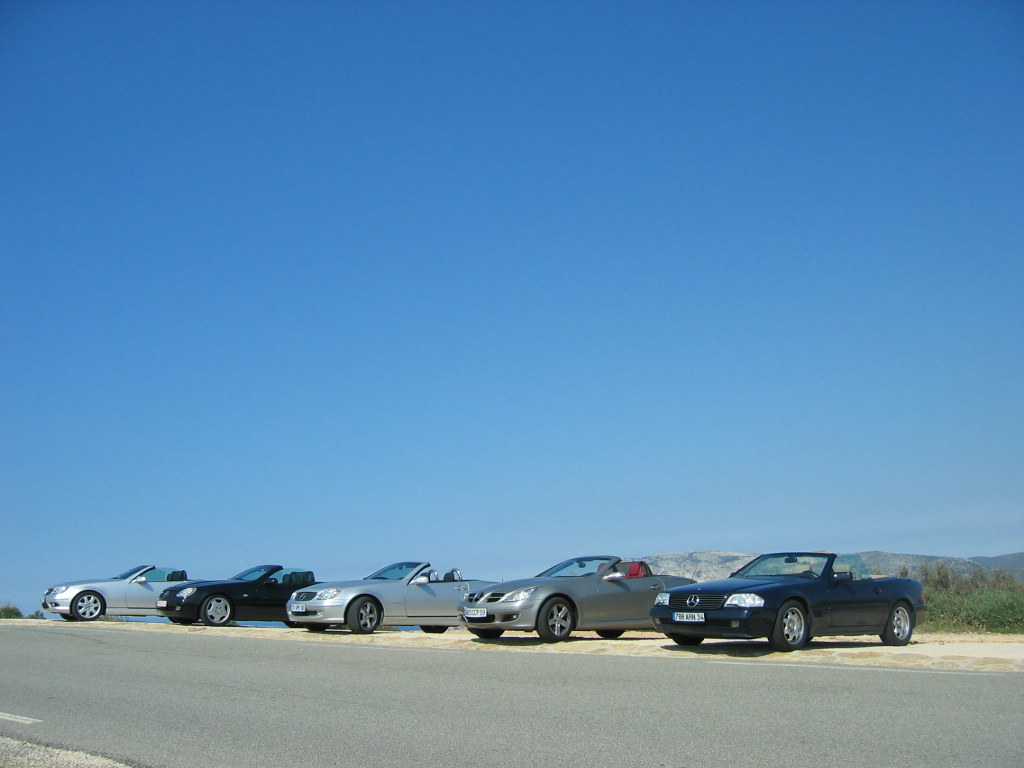Here is a detailed caption combining the key points from both descriptions:

In this photograph, five Mercedes convertible cars are lined up on the side of a gray, concrete-paved road that cuts through a desert-like landscape. The first car, closest to the foreground on the right, is a dark navy blue Mercedes with a white license plate that starts with the number 7. Following it are two silver Mercedes: the first with red seats and the second with black seats. The fourth car is either a dark blue or black Mercedes, and the line-up concludes with another silver Mercedes. These cars are neatly parked in a stretch of light tan or almost white sand adjacent to the road. To the right side of the composition, a scattering of green bushes can be seen. In the far background, the landscape is framed by mountains. Dominating the top three-quarters of the image is an expansive, clear blue sky, creating a striking contrast with the arid terrain below.